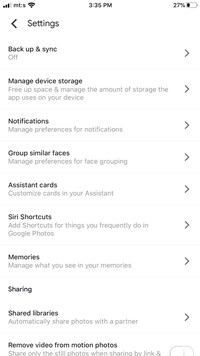This image depicts a cell phone screen displaying the 'Settings' menu of a mobile application. The background is white, and standard cell phone status icons are visible at the top. On the left, signal strength bars are displayed, indicating cellular reception. In the center, the current time reads "3:35 PM." On the right, a horizontal battery icon shows a remaining charge of 27%.

Below the status bar, the screen features a header with a left-facing arrow and the word "Settings" in larger type. Directly beneath the header, in bold black type, is a list of 10 settings options, each accompanied by a right-facing caret indicating that the user can select it for further customization.

The settings options are as follows:

1. **Backup & Sync:** Currently set to "Off."
2. **Manage Device Storage:** Described as "Free up space and manage the amount of storage the app uses on your device."
3. **Notifications:** Described as "Manage preferences for notifications."
4. **Group Similar Faces:** Described as "Manage preferences for face grouping."
5. **Assistant Cards:** Described as "Customize cards in your assistant."
6. **Siri Shortcuts:** Described as "Add shortcuts for things you frequently do in Google Photos."
7. **Memories:** Described as "Manage what you see in your memories."

The following option, **Sharing**, acts as a category header under which two sub-options are listed:

8. **Shared Libraries:** Described as "Automatically share photos with a partner."
9. **Remove Video from Motion Photos:** Described as "Share only the still photos when sharing a link," though the rest of this description is cut off at the bottom of the screen.

Each setting option is designed to be easily accessible, allowing users to customize and manage various aspects of their app experience effectively.